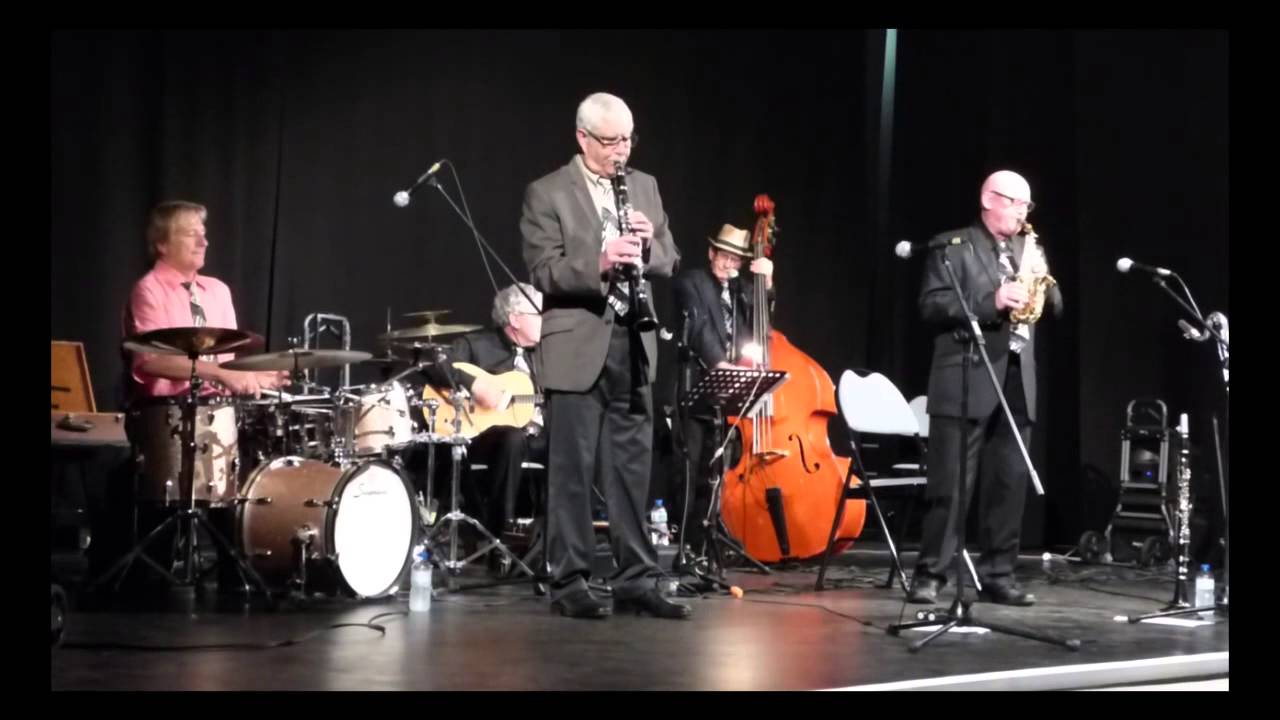This photograph captures an older, five-member band performing on stage, all dressed in black suits except for the drummer, who is distinctive in his pink dress shirt and tie. Positioned against a backdrop of black curtains, the stage itself is also black and framed by a black border. At the front and center, a man with glasses plays a clarinet, while to his left, another bespectacled man skillfully handles a saxophone. The saxophone player is bald, and the clarinet player appears focused on his performance. Behind them, a man wearing a tan top hat plays the cello, adding depth to the arrangement. Centrally located is a guitarist playing an acoustic guitar, and to the far left, the drummer—who stands out due to his unique attire—keeps the rhythm on a tan drum set. Additional elements on the stage include several microphones on stands, folding chairs, and other musical equipment. The ambiance is professional and classic, with an evident emphasis on the detailed and harmonious ensemble.